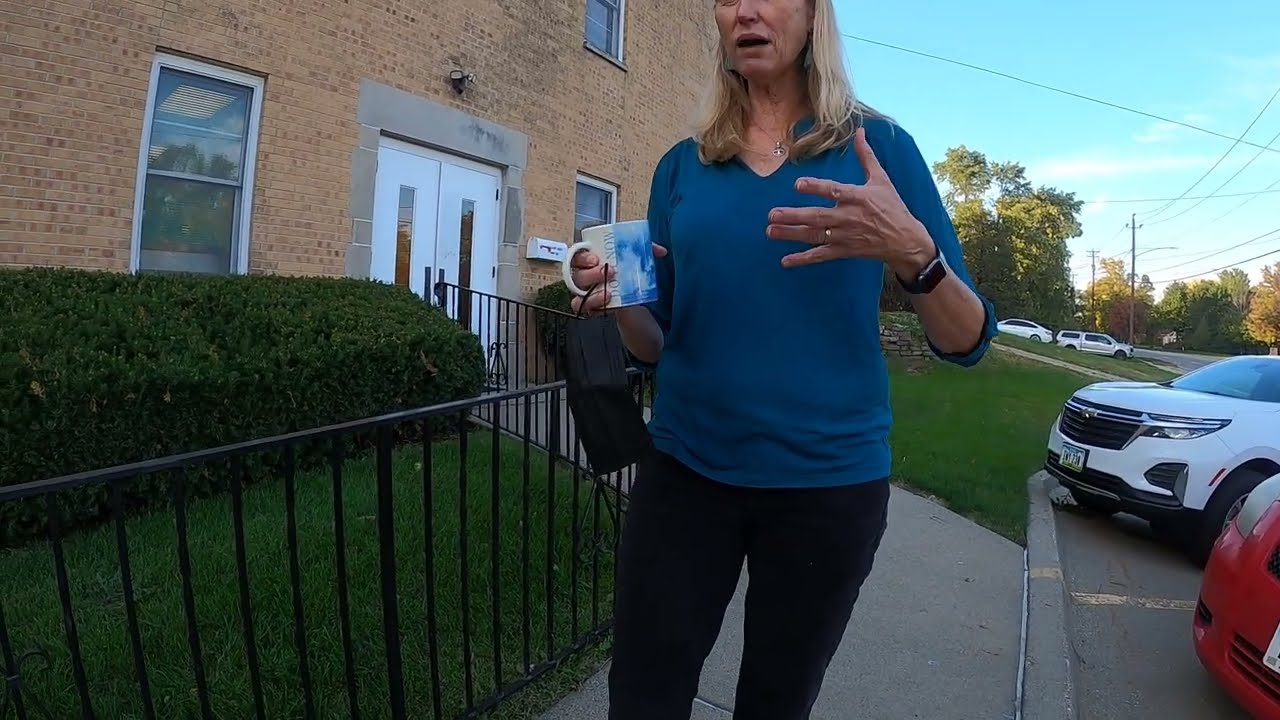A middle-aged Caucasian woman with shoulder-length blonde hair stands on a sidewalk in front of a large brick building, possibly a school or apartment complex. She is wearing black pants and a blue V-neck shirt, accessorized with an Apple Watch and a gold wedding ring on her left hand. She holds a white mug with a blue design in her right hand and her left arm is extended outward, suggesting she is engaged in conversation, possibly during a television interview. The woman's mouth is open, and her expressive posture indicates she is explaining something. A black fence with a manicured bush and green grass stands behind her, along with multiple windows and a door on the brick building. To her right is a parking lot with a white SUV and a red car partially visible. Additional background elements include more cars, a street, telephone poles, and trees.